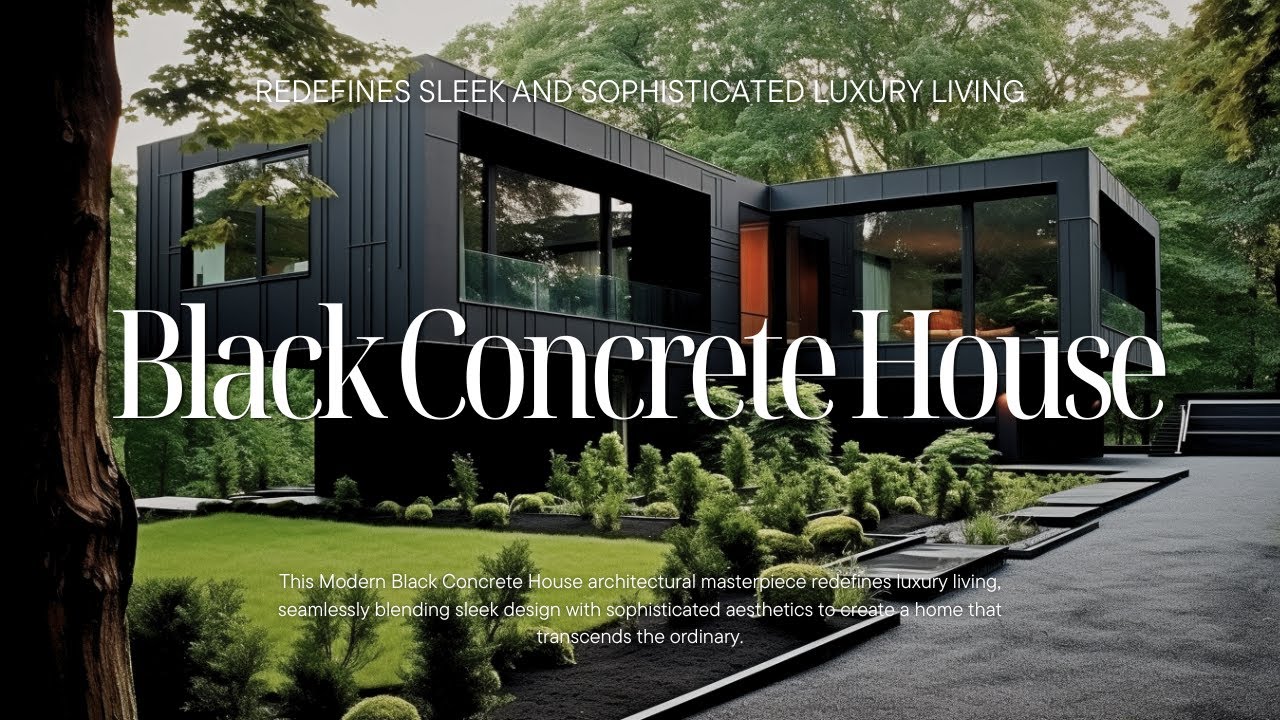The image serves as a visually striking advertisement for the "Black Concrete House," showcasing a modern architectural masterpiece. The central focus is bold white text proclaiming "Black Concrete House, the irony," surrounded by a visually captivating black house. This house exudes modernity with its sleek design, characterized by an abundance of large windows that invite natural light and create a sense of openness. The structure itself comprises smooth surfaces and sharp right angles, giving it a distinct geometric aesthetic. The top of the image features the tagline in white text: "Redefine Sleek and Sophisticated Luxury Living," emphasizing the house’s avant-garde elegance. Nestled in a wooded area with beautifully landscaped surroundings, the house features a grey slate patio and appears to consist of two prominent rectangular sections. Some windows are described to be electrically operable, adding a touch of futuristic convenience. Low planter beds with black chips and minimalist vegetation complement the design, while a striking red door and black asphalt driveway add contrast. The large white text at the bottom praises the house as a modern architectural marvel, stating: "This modern black concrete house architectural masterpiece redefines luxury living, seamlessly balancing sleek design with sophisticated aesthetics to create a home that transcends the ordinary." The overall presentation captures a sense of secluded luxury, ideal for those seeking an elegant and private living space.